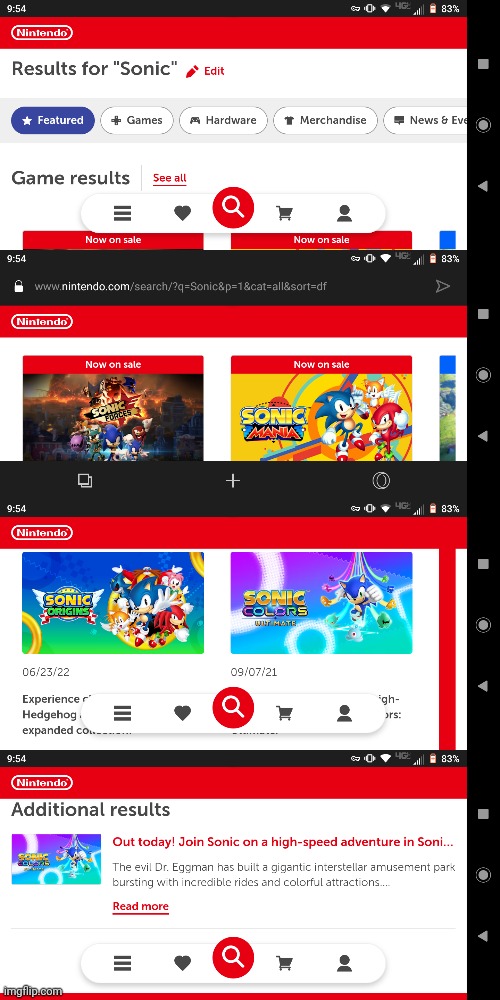This composite image features four sequential screenshots captured on a mobile phone from the Nintendo website. Each screenshot is stacked vertically, creating a rectangular collage.

In the first screenshot, the user has searched for "Sonic" on the website. The second screenshot reveals two Sonic franchise games: "Sonic Forces" and "Sonic Mania." Moving to the third screenshot, two additional Sonic games are displayed: "Sonic Origins" and "Sonic Colors." The final screenshot prominently showcases a promotional section titled "Additional Results." Here, the text invites players to join Sonic on a high-speed adventure, battling the evil Dr. Eggman in a colossal interstellar amusement park filled with remarkable rides and vivid attractions. The text also mentions the option for users to read more about these offerings.

Overall, this detailed visual captures a thorough exploration of Sonic-related content on the Nintendo website through a series of mobile phone screenshots.